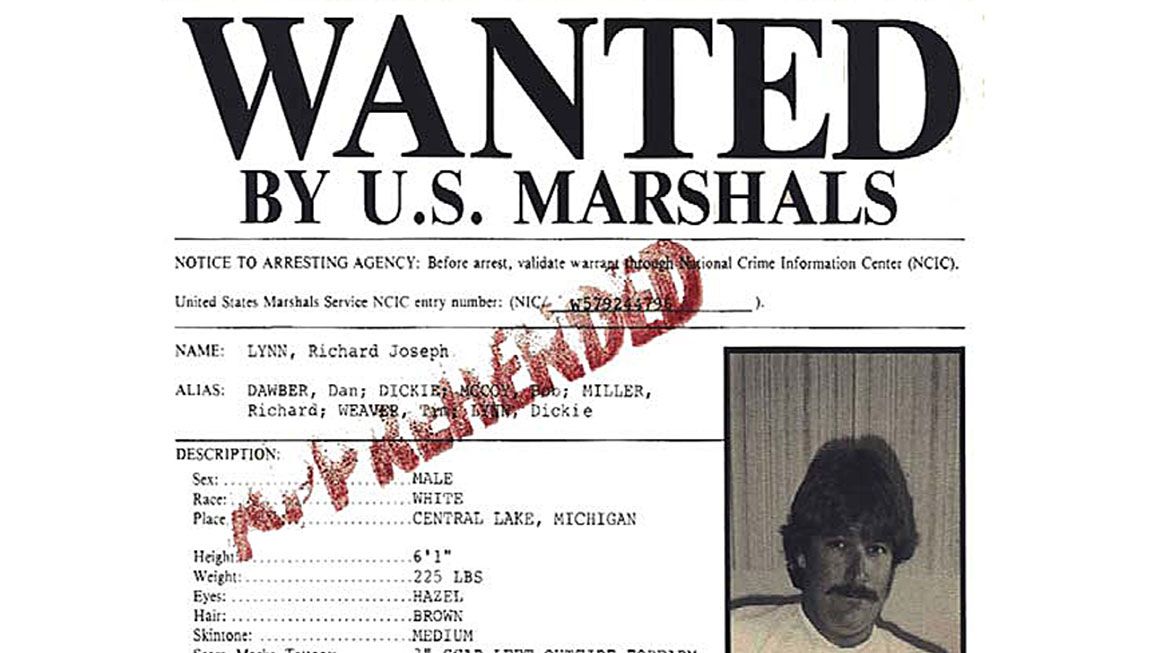This image depicts a wanted poster issued by the U.S. Marshals, which appears to have been digitally enhanced, as indicated by the unusually bright white background suggestive of photo editing. The poster features a black-and-white photograph of the suspect, a white male with dark hair and a mustache, framed by a black border. The photograph has a slightly worn stamp across it, indicating the word "APPREHENDED."

The text on the poster begins with "WANTED BY U.S. MARSHALS" in large, bold letters, followed by a notice to arresting agencies advising to validate the warrant through the National Crime Information Center (NCIC).

The suspect is identified as Richard Joseph Lynn, with aliases listed as Dauber, Dan, or Dickie. Detailed physical descriptions are provided: he is a white male from Central Lake, Michigan, standing 6'1" tall, with brown hair, hazel eyes, and weighing approximately 225 pounds.